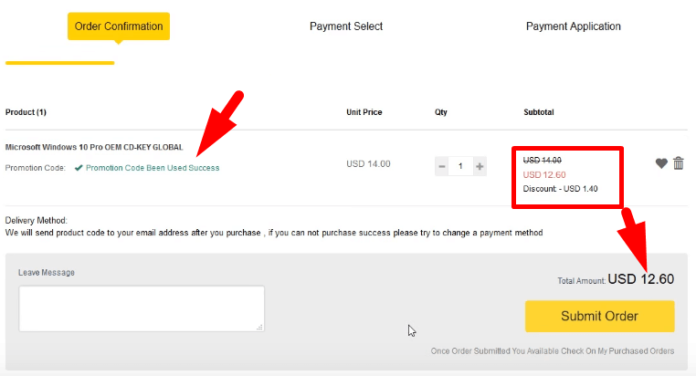This image is a rectangular screenshot of an order confirmation page from an e-commerce platform. At the top of the page, there are three sections labeled "Order Confirmation," "Payment Select," and "Payment Application." The "Order Confirmation" section is highlighted in yellow, indicating that the user is currently on this page.

In the main body of the page, the details of the purchase are clearly displayed. The product being bought is "Microsoft Windows 10 Pro (Key - Global)." The pricing details are broken down into unit price, quantity, and subtotal. The unit price for the product is USD $14, with a quantity of 1, resulting in a subtotal of $14.

A promotional code has been successfully applied, as indicated by a red arrow, which provided a discount of $1.40. This results in a total amount of USD $12.60, highlighted in a red rectangle with an arrow pointing to it for emphasis.

At the bottom of the page, there is a large yellow button labeled "Submit Order," indicating that the purchase has not yet been finalized.